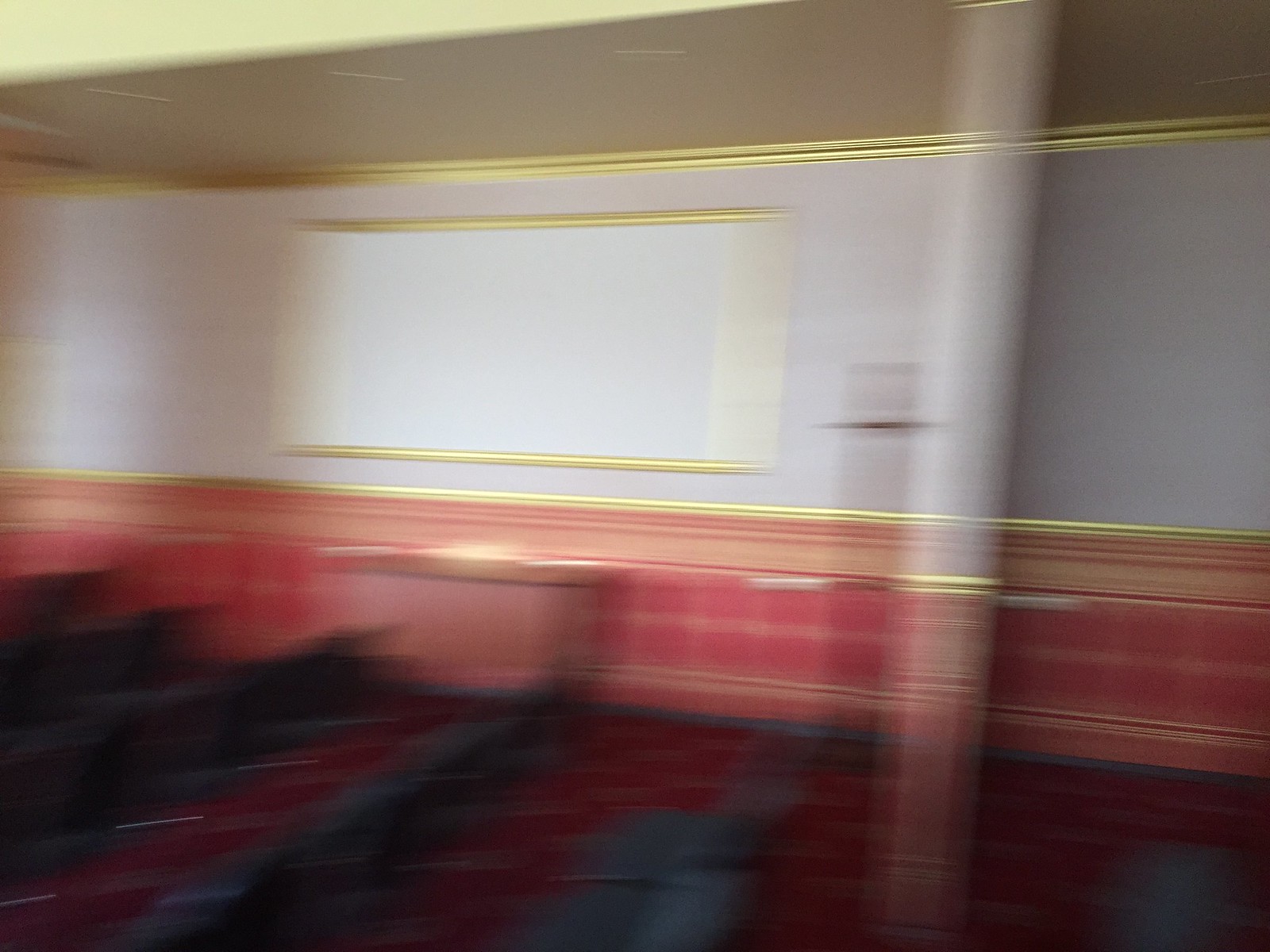This hastily captured image, although blurry, portrays a room with a distinctive decor. Dominating one wall is a whiteboard, outlined with a golden trim at both the top and bottom edges. The wall itself follows a similar pattern; the upper section is white with golden borders running along the top and bottom, while the area closer to the floor transitions to a peach color, adding a warm contrast. A white post is visible within the room, contributing to the structural layout. Scattered across the main floor are several benches, suggesting this space might be utilized as a conference room.